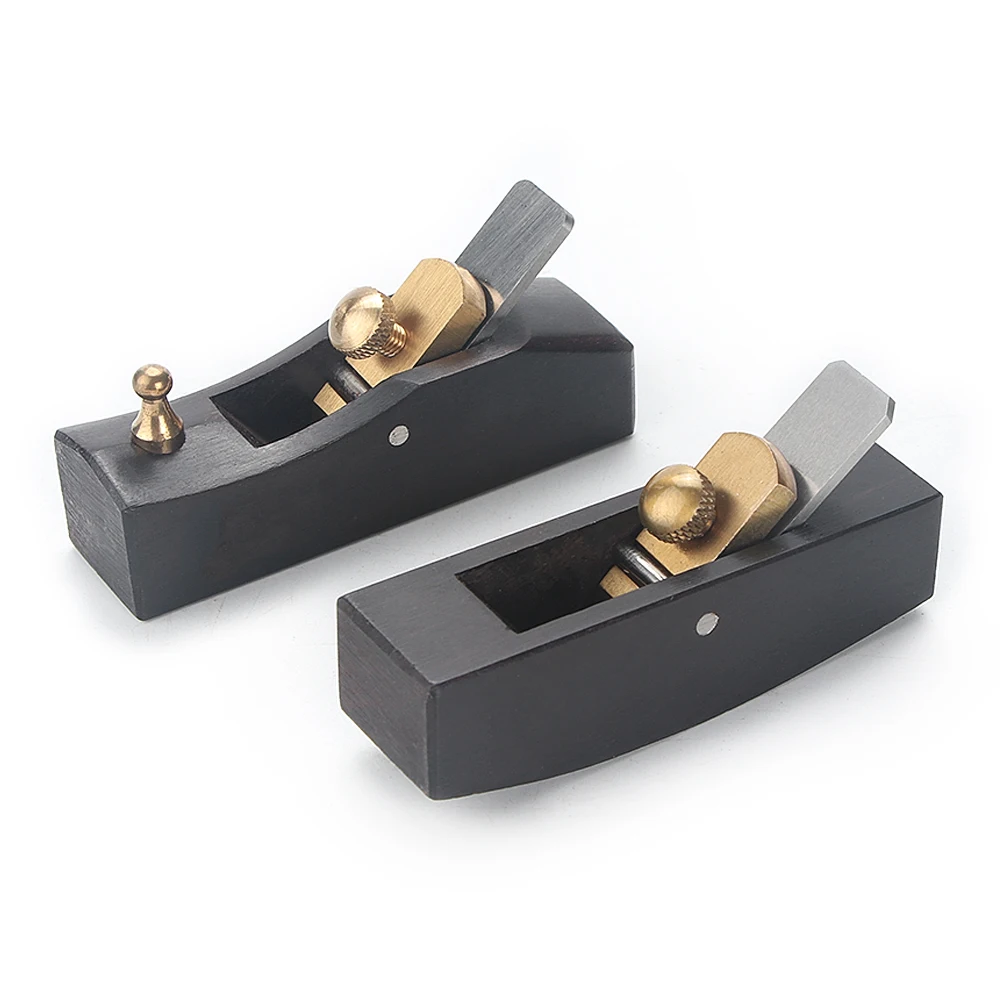In the image, we see two finely polished metal tools against a white background, illuminated from the upper left. The tools, made of a combination of brass and steel, are positioned with one at the top left and the other at the bottom right of the image. The tool on the top left features a distinctive metallic knob that resembles a pawn piece from a chess set, mounted on its black body, which is flat on the bottom. This knob is set on a revolving brass piece. In contrast, the tool on the bottom right lacks this knob, instead featuring a semicircular base that allows it to rock back and forth. Both tools show intricate details, including metallic knots on the right side where the handle attaches to the main body and flat surfaces supporting the handles. The design differences between the two tools suggest distinct functionalities, even though their exact purpose remains unclear.